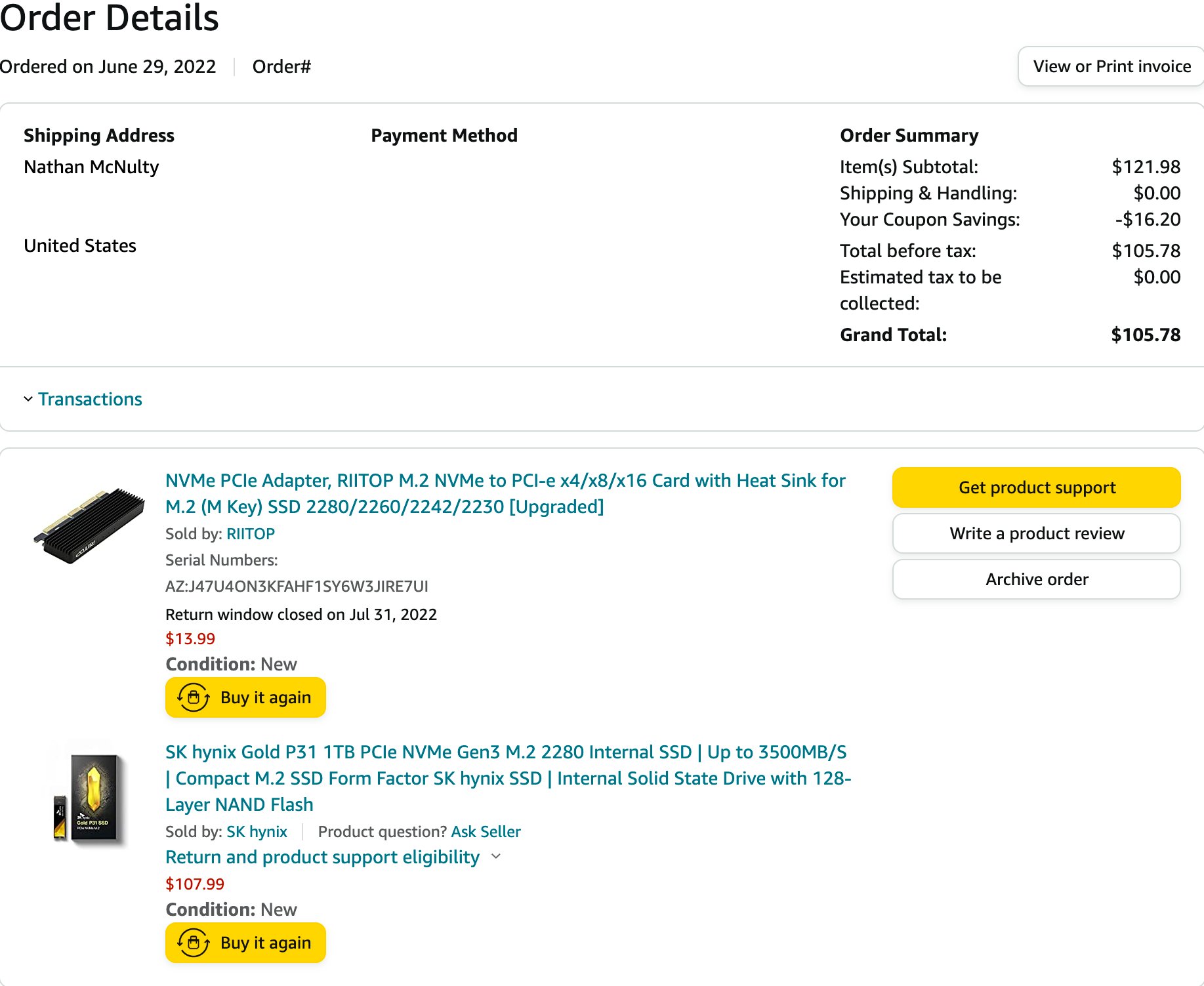The image displays a detailed view of an Amazon Order Details page. In the top left corner, prominently, it reads "Order Details," with a secondary occurrence positioned below it in smaller font. The order was placed on June 29, 2022, but the order number is not visible. On the far right, there's a button labeled "View or Print Invoice" for accessing the invoice.

A horizontal line delineates the "Ordered On" section from the "Shipping Address" section. The shipping address is bolded and lists "Nathan McNutty" in the United States, with a blank space below for the payment method.

Under "Order Summary," the item subtotal is stated as $121.98, with shipping and handling costs at $0.00. The coupon savings are listed as $16.20, reducing the total before tax to $105.78. There is no estimated tax, making the grand total $105.78, which is bolded.

The image includes an expandable "Transactions" section in blue, as well as two itemized products with thumbnails. The first item is an upgraded NVME adapter sold by a specific seller, with a serial number listed as a combination of letters and numbers. The return window for this item is open until July 31st, and it is priced at $13.99. Options include buying it again, accessing product support, writing a product review, or archiving the order.

The second item listed is an internal SSD priced at $107.99, with a similar set of options for managing the purchase.